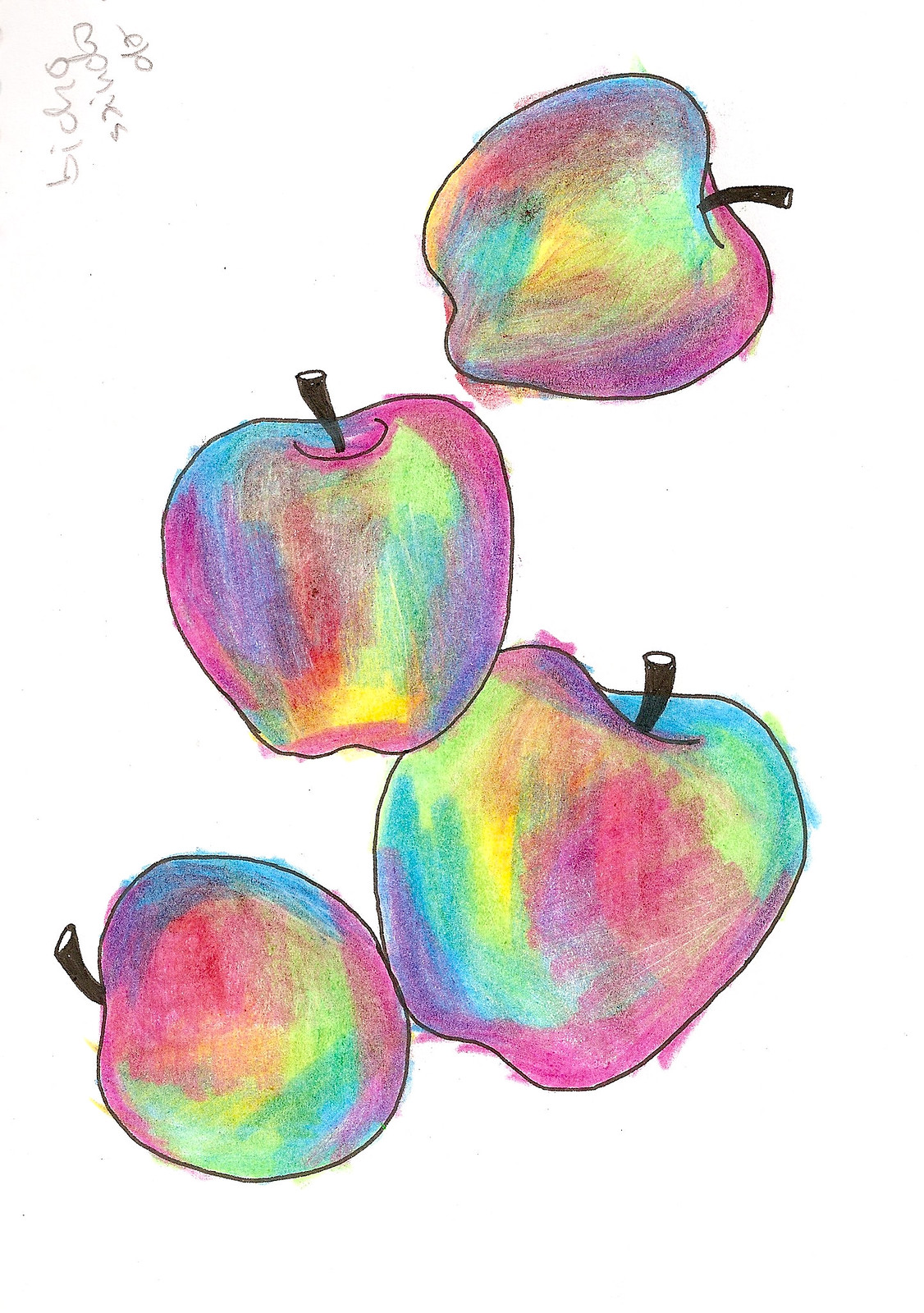This artwork is an imaginative and colorful illustration of four apples, each decorated in a vibrant array of rainbow hues including shades of pink, purple, yellow, green, blue, and red. The apples are bordered with thick black outlines, giving them a coloring book appearance, and appear to have been filled in with crayons or colored pencils, with colors artistically spilling outside the lines. One apple, situated sideways with its stem pointing to the right, is located near the top right corner. Two smaller, similarly sized apples are positioned above the largest apple which sits prominently in the bottom right corner. The smallest apple, touching the largest, is turned leftward. The stems of the apples are drawn in black, tipped with white. The background is plain white, without any borders, enhancing the array of colors of the apples. In the top left corner, there is a signature or marking that appears to be penned in pencil, though it is difficult to decipher, possibly reading "bicho" or something similar. The entire composition of the apples seems as though they are almost stacked or falling in a semi-random arrangement, adding a dynamic quality to the piece.